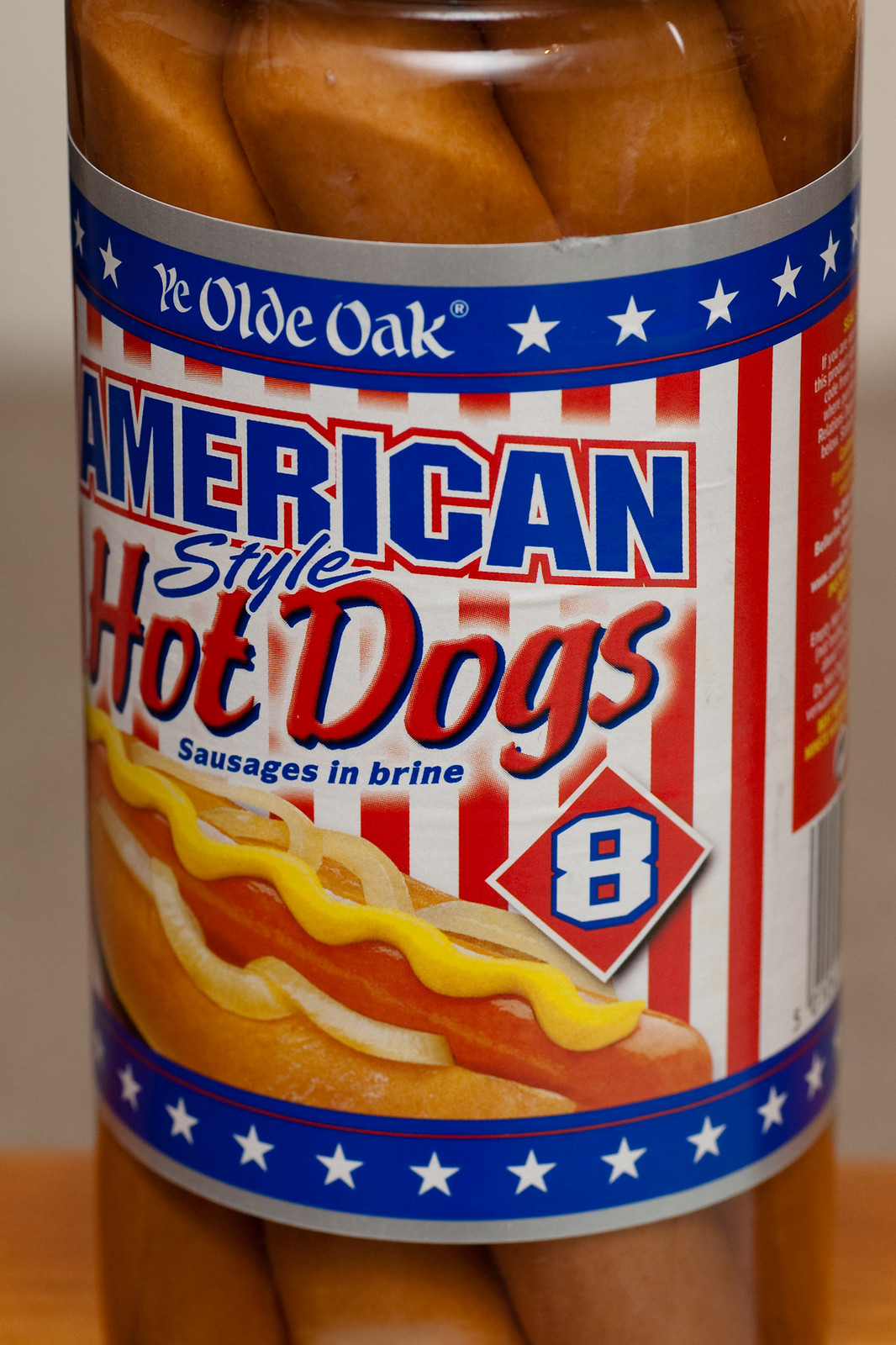This close-up photograph, in a rectangular portrait orientation, captures a jar of food prominently. The label at the top displays "Ye Olde Oak" in a white font set against a blue background adorned with white stars. Below, the words "American Style" are presented in a bold blue font, followed by "Hot Dogs" in striking red. Further down, "Sausages in Brine" is written in blue font. The label also features an appetizing image of a hot dog topped with a line of yellow mustard. Through the glass of the jar, light brown hot dogs are visible. The background of the image transitions between white and light orange hues, providing a subtle and warm backdrop for the subject.